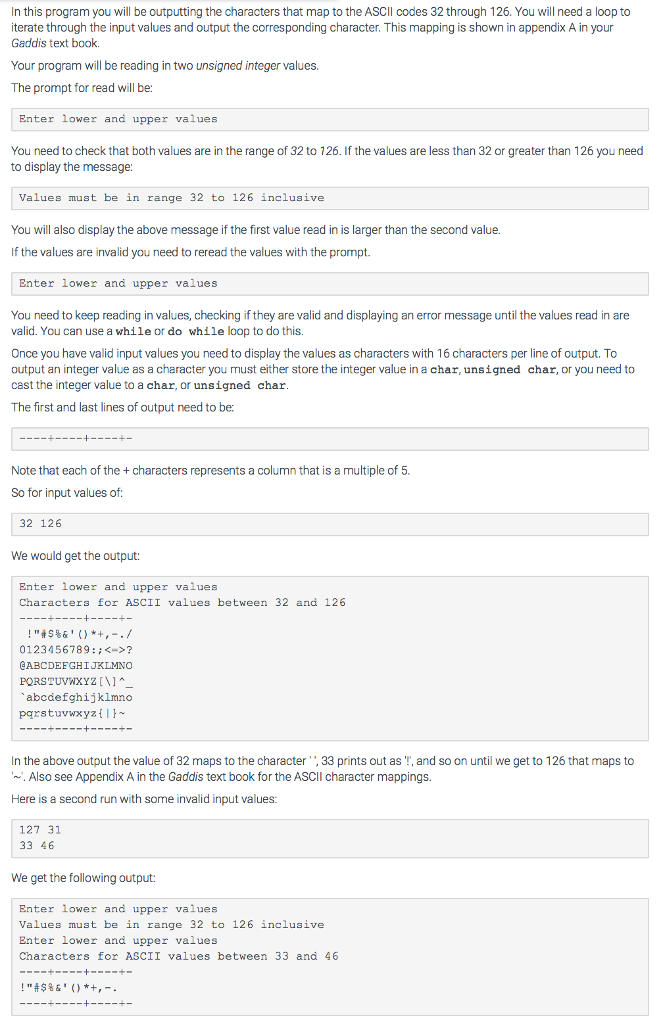**Screenshot of Computer Coding Informational Page**

This screenshot showcases an educational web page focused on teaching basic computer programming concepts. The page features a clean, white background with small, black text, and includes a few light gray bars to highlight headings.

The main content describes a coding exercise in which the user is required to output characters corresponding to ASCII codes ranging from 32 to 126. The instructions specify that a loop must be used to iterate through the input values and produce the corresponding characters. Details on the ASCII character mappings are referenced in Appendix A of the GADIS textbook.

The program expects two unsigned integer inputs, as indicated by a prompt presented within a gray box: "enter lower and upper values." Overall, the page appears to serve as a teaching aid or informational guide for beginners learning about computer coding.